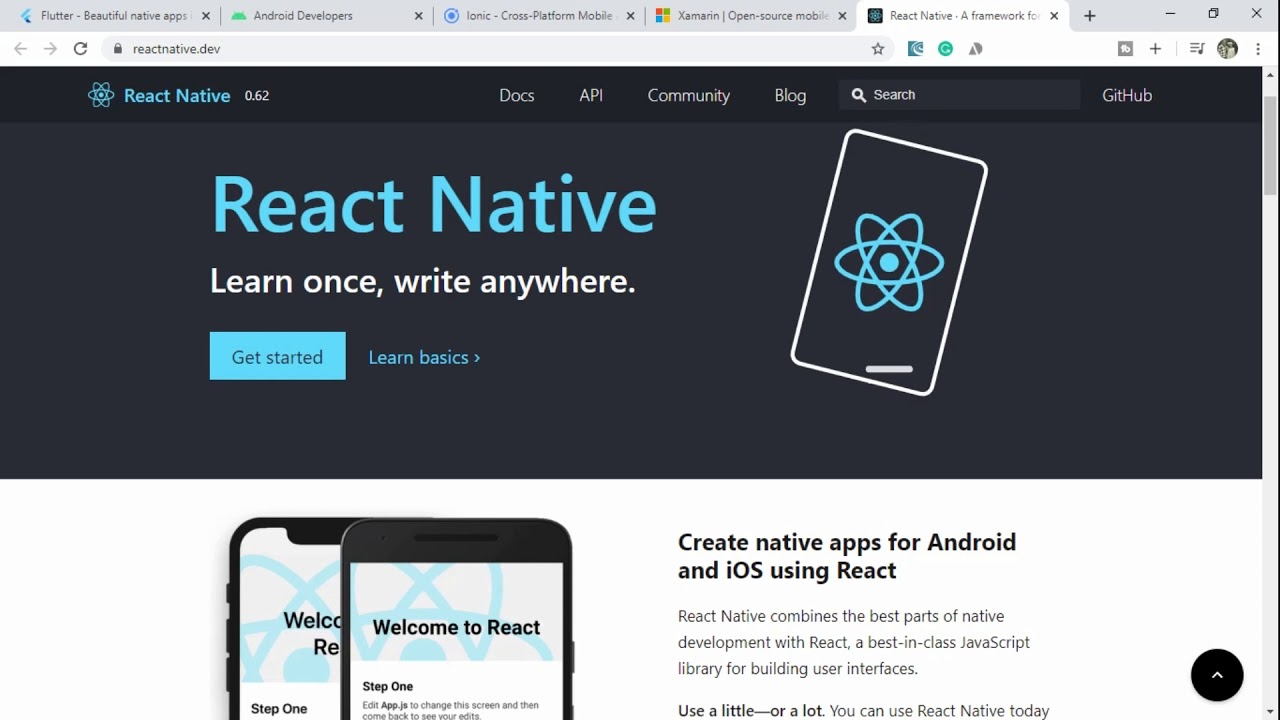The image features a user interface on a white background, with a prominent blue outline along the top and right side. On the right, there is a vertical scrollbar. Along the top, a series of blue tabs display small icons, including a blue icon, a green icon, a blue circle, a multicolored box, a white icon, a blue icon with a plus and minus sign, some page icons, an X icon, left and right arrows, and a circular refresh icon. Further to the right, there's a search box, followed by a blue square and blue circle, a gray cone-shaped icon, a little square with a plus sign, a square with a blue circle, a small gray circle, and an icon with three dots.

The central part of the interface features a black background that displays text "React Native 0.62", accompanied by a blue atom icon. At the top of the black section are the menu options: Docs, Apps, Community, Blog, Search, and Gift Hub.

Within the black box, there is text in blue that reads "React Native" and below it, in white text, "Learn Once, Write Anywhere". A blue "Get Started" button and a blue "Learn Basics" button are also visible. Below these buttons is an image of a white phone displaying the blue atom icon, with a small white mark at its bottom.

Descending further, a white box shows two black phones labeled "Welcome to React, Step 1", along with the messages "Create Native Apps for Android and iOS using React" and "Use a Little or a Lot". At the very bottom of the image, a small black circle with an up arrow is present.